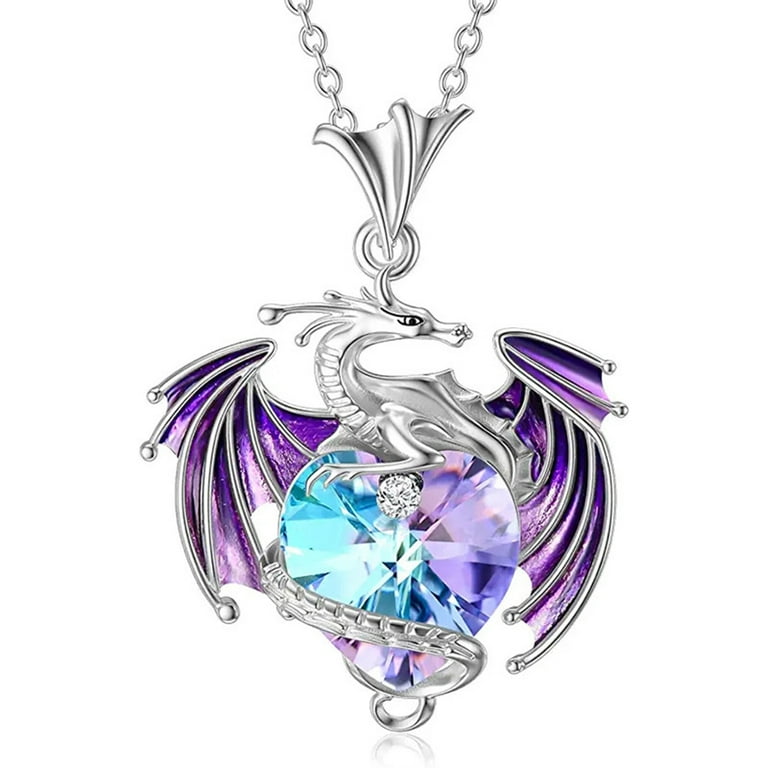The image showcases a detailed silver necklace, prominently featuring a dragon pendant. The dragon, crafted with visible scales and outlined eyes, has its wings spread out and colored in vibrant purples. Its tail wraps protectively around a heart-shaped crystal, which glimmers in shades of blue, pink, and purple. The centerpiece of the heart crystal boasts a shining diamond. The entire pendant, which appears to be made of sterling silver, hangs from a matching silver chain. The necklace exudes elaborate craftsmanship, with intricate detailing on both the dragon and its wings. The background is a pale white, allowing the vivid colors and intricate details of the pendant to stand out prominently.